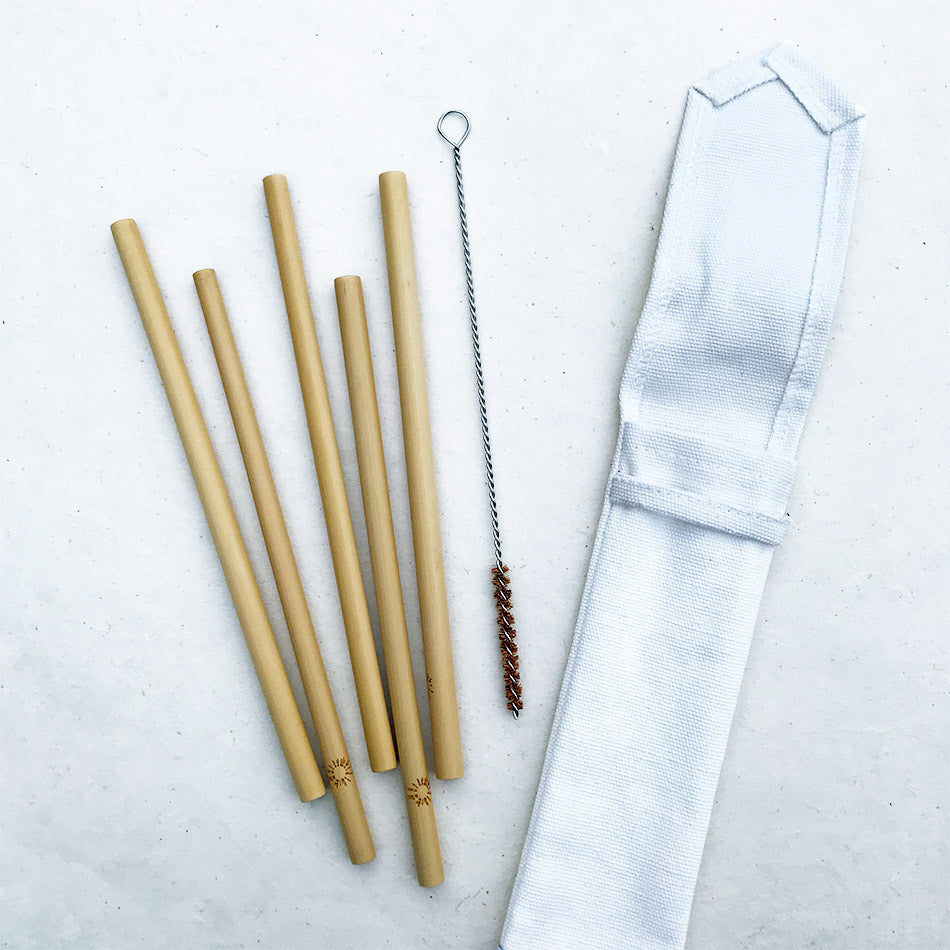The image depicts an overhead view of a product set displayed on a white background. On the left side, there are five wooden, dowel-shaped objects approximately the size of straws, each adorned with a small sun engraving. These objects are made of light wood and are likely hollow. Beside them is a metal wire brush, featuring brown bristles and a twisted silver handle with a loop on one end, designed for cleaning the wooden pipes. To the right of the brush, there is a white canvas pouch with a pointed top and a single loop for closure, intended for storing and carrying the wooden dowels and the cleaning brush.